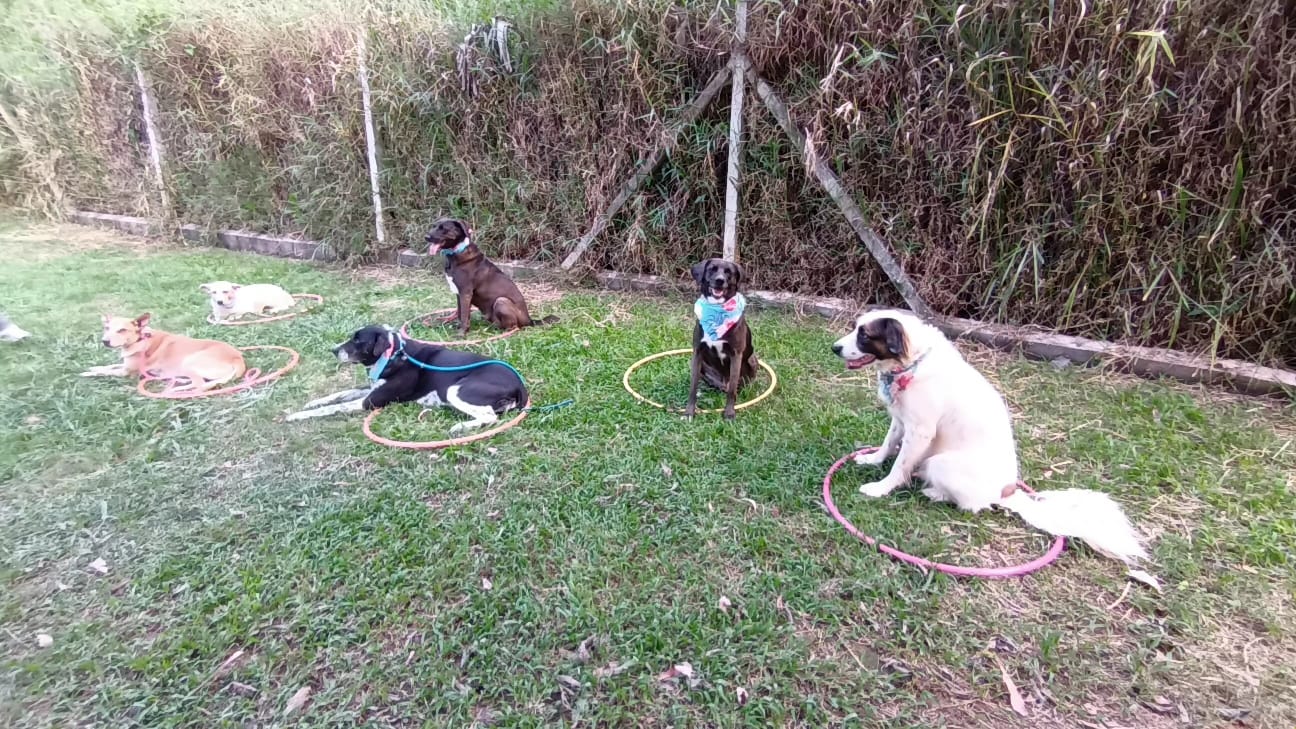This is a color photograph taken outdoors during clear weather, depicting six medium to large-sized dogs of various breeds and colors seated and lying down in individual hula hoops on a grassy field. The grass is somewhat dry and patchy in places. Three of the dogs are sitting, and three are lying down inside pastel-colored, worn-looking hula hoops. From left to right, the dogs are positioned as follows: a brown dog sitting in a yellow hula hoop, with a white dog lying down slightly behind in another hoop; a black and white dog sitting in a worn light-colored hoop with a brown dog wearing a bandana sitting behind in another hoop; a brown dog with its tongue hanging out sitting in a hula hoop in the next row, facing directly at the viewer, the only one doing so; and lastly, towards the right, a mostly white dog with brown facial markings and a fluffy tail seated in a pink hula hoop, also facing left. Behind the dogs is a wire fence supported by weathered wooden posts. Beyond the fence, tall grasses, shrubs, and brush form a dense, natural barrier, giving the appearance of a plant wall. The overall scene suggests an organized outdoor dog training activity or obedience class.